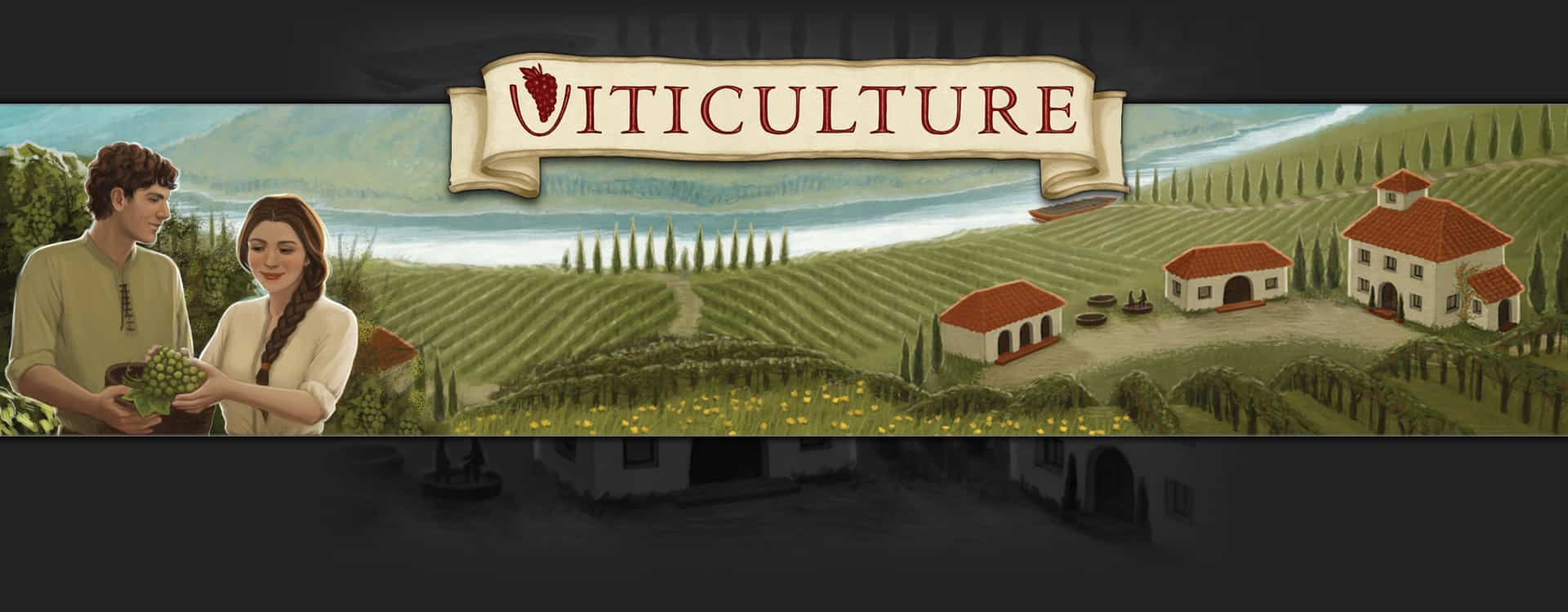This detailed and organized illustration presents a vibrant landscape of a vineyard with picturesque rolling hills. On the right side of the image, three Spanish-style buildings with red tile roofs stand prominently. The largest of these buildings is two stories high, accompanied by two smaller structures. Neatly arranged rows of grapevines stretch across the scene, denoting a well-maintained vineyard. Beyond the buildings, a flowing river winds through the landscape, featuring a dock or barge near its shore. Across the river, additional fields extend into the distance, though their details fade into the horizon. On the left, a couple is depicted harvesting green grapes, placing them into a basket. The woman is characterized by her braided brown hair and white shirt, while the man is dressed in a green shirt and has curly hair. Above this pastoral scene, a beige banner with rippled ends reads "VITICULTURE" in red capital letters, with a bunch of grapes artistically integrated into the "V."